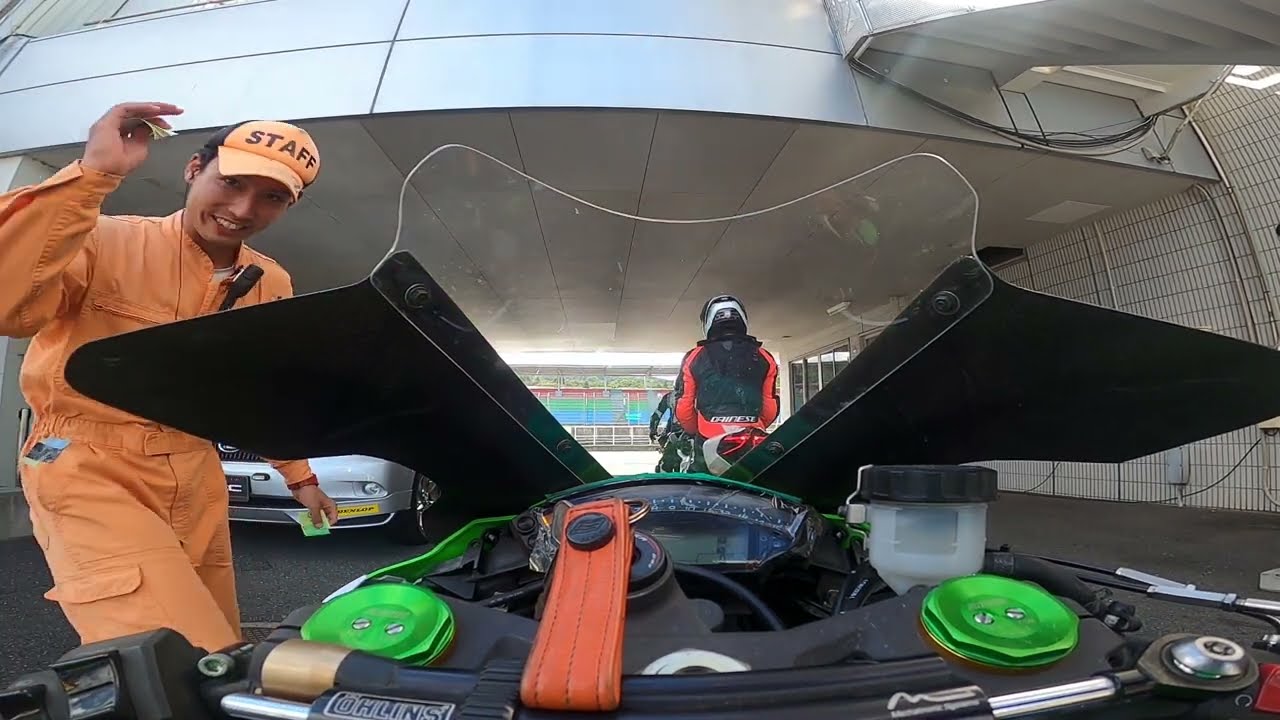This horizontal, rectangular photograph captures a scene likely set in a maintenance or pit crew area, possibly at a racing event or motorcycle repair shop. Dominating the image is a vehicle that seems to be a motorcycle, identifiable by its open compartment and visible motor adorned with green components, orange strips, and various hoses. The vehicle appears to have a windshield with black areas and a translucent upper section.

On the left side of the image stands a man in a light orange jumpsuit and matching hat labeled "staff," suggesting his role as part of a pit crew. He is smiling and appears to be stepping towards or working on the motorcycle. In the background, there is another individual sitting on a motorcycle, donned in a black jacket with red stripes and a black helmet featuring a white stripe. He seems to be parked in front of a bench, and behind them, concrete structures hint at the setting being an industrial or parking lot area.

Above and beyond this main interaction, a building with light blue reflective surfaces and white walls stretches across the upper part of the image. The building's metallic, roundish architecture reflects the blue sky, lending a structured yet open feel to the environment.